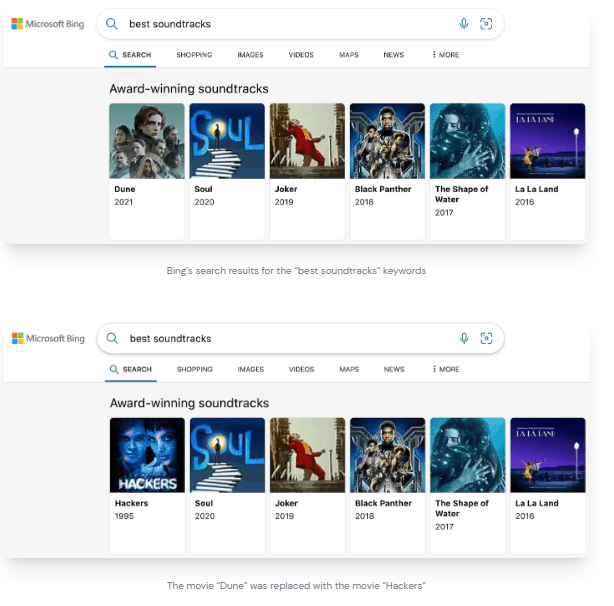This image features two side-by-side screenshots sourced from Microsoft Bing. Both images display identical search results for the term "best soundtracks" in Bing's search interface. The top screenshot showcases the older Microsoft Bing logo, consisting of the traditional four-colored Windows icon (green, red, blue, and yellow) and the "Microsoft Bing" name in gray font on a white background. The search box appears as a rectangular shape with rounded corners, containing the search term "best soundtracks" in gray font.

The search results begin with a headline reading "Award-winning soundtracks" and present images from five different movies, all displayed from left to right. The listed movies and their corresponding years are: "Dune" (2021), "Soul" (2020), "Joker" (2019), "Black Panther" (2018), and "The Shape of Water" (2017), with "La La Land" (2018) displayed on the far right.

The second screenshot, located directly beneath the first, is visually identical except for the inclusion of additional text in gray font interspersed with white space. The text states, "Bing search results for the best soundtracks keywords." On closer inspection, the only variation between the two screenshots becomes apparent: in the second image, the movie "Dune" has been replaced with "Hackers" (1995) on the far left, while the rest of the search results and their associated visuals remain the same.